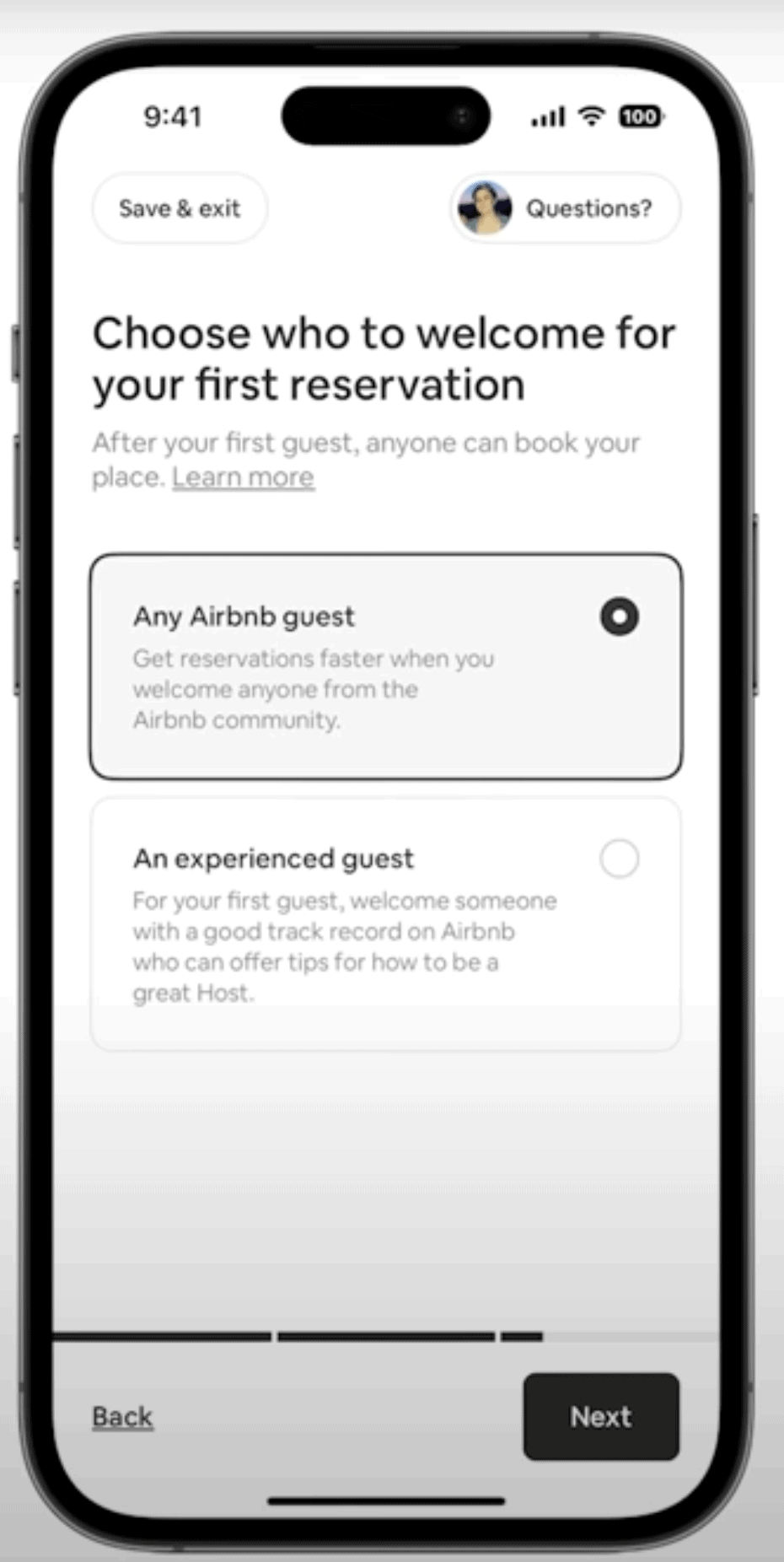A close-up view of a smartphone screen is captured, revealing the phone's borders, and showcasing the power button on both the left and right sides. The screen displays the time as 9:41, with Wi-Fi connectivity and a fully charged battery icon at 100% on the right. Below the time on the left side, there is a "Save and Exit" button, while on the right, an icon of a person next to the word "Questions" is displayed. Dominating the center of the screen in large font is the text: "Choose who to welcome for your first reservation." Beneath this, smaller text explains, "After your first guest, anyone can book your place," followed by a "Learn More" link. Two interactive buttons are visible below this section. The top button, labeled "Airbnb guest," encourages users to "Get reservations faster when you welcome anybody from the community." The second button, labeled "Experienced guest," suggests welcoming "somebody with a good track record on Airbnb" for the first booking. At the bottom of the screen, a status bar runs in black, housing a "Back" button on the left and a black "Next" button on the right. The background of the screen is predominantly white.